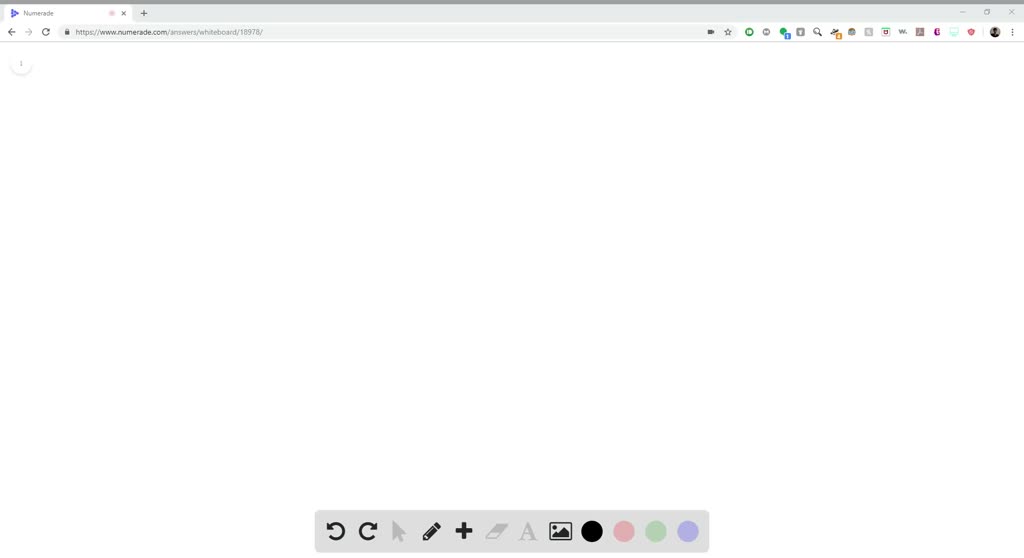A detailed caption for an image of the described screen could be:

"The screen displays a blank interface with various menu elements. At the top, a thin gray bar runs horizontally across the screen. On the left-hand side of this bar, there's a tab featuring a purple triangle pointing right, likely labeled 'Numerals,' adjacent to a yellow star with an ‘X.’ Afterward, the bar continues in gray, displaying a plus sign in the middle. Toward the far right, there are icons for minimizing (dash), restoring (two stacked boxes), and closing (X) the window.

Beneath the gray bar, a white bar features navigation icons including a dark gray left arrow, a lighter gray right arrow, and a circular refresh icon. Within an oblong shape on this bar, there is a URL (too small to read), ending with an icon and an open star. There are also fifteen other small icons distributed along this line, culminating at the far right with three vertical dots indicating additional options.

The main body of the interface is a white blank space, followed by another gray toolbar loaded with various tool icons. These include two circular arrows for refreshing (one pointing right and the other left), an up-pointing arrow, a pencil icon for editing, and a plus icon for adding new elements."